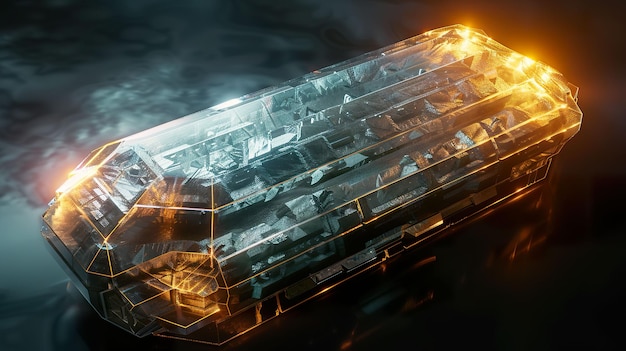The image appears to depict a computer-rendered, space-age contraption that resembles a large, cube-like vehicle with rounded corners. It has multiple stories or sections: a bottom, middle, and top, but lacks a traditional captain's nest. Its structure is clear and transparent, allowing visibility of the internal mechanics that feature silver and aluminum foil elements. The exterior is illuminated with bright yellow and golden lights at both ends, creating a striking contrast against the dark aqua, dark blue, and dark brown hues that dominate its design. The lights and materials give it a futuristic, almost otherworldly appearance, evocative of technology found in outer space narratives. The contraption is set against a backdrop that transitions from a slate blue, cloudy color on the left to a stark, black surface on the right, enhancing its mysterious and advanced aesthetic.